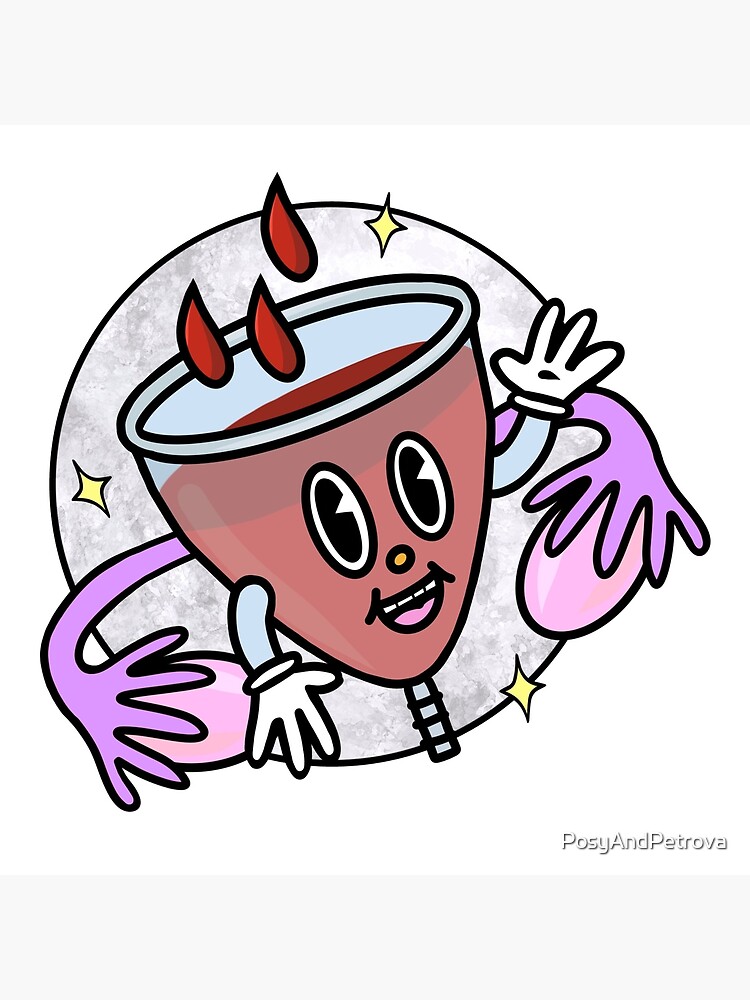The cartoon graphic displays a smiling cup with expressive eyes and a yellow nose, filled with a red liquid that appears to be blood. The cup has two arms, one raised and one by its side, with hands resembling gloves. The background is white, and in the bottom right, it reads "Posey and Petrova," likely the artist's signature. The cup is integrated within a circular design which also features symbolic elements of the female reproductive system: purple fallopian tubes extending like arms, holding pink ovaries. Above the cup, three large drops of red liquid are dripping into its open top. Decorative stars surround the cup, adding to the whimsical and lighthearted aesthetic. This image seems to be a playful and artistic representation of menstruation, possibly emphasizing themes related to women's periods and Mother Nature.